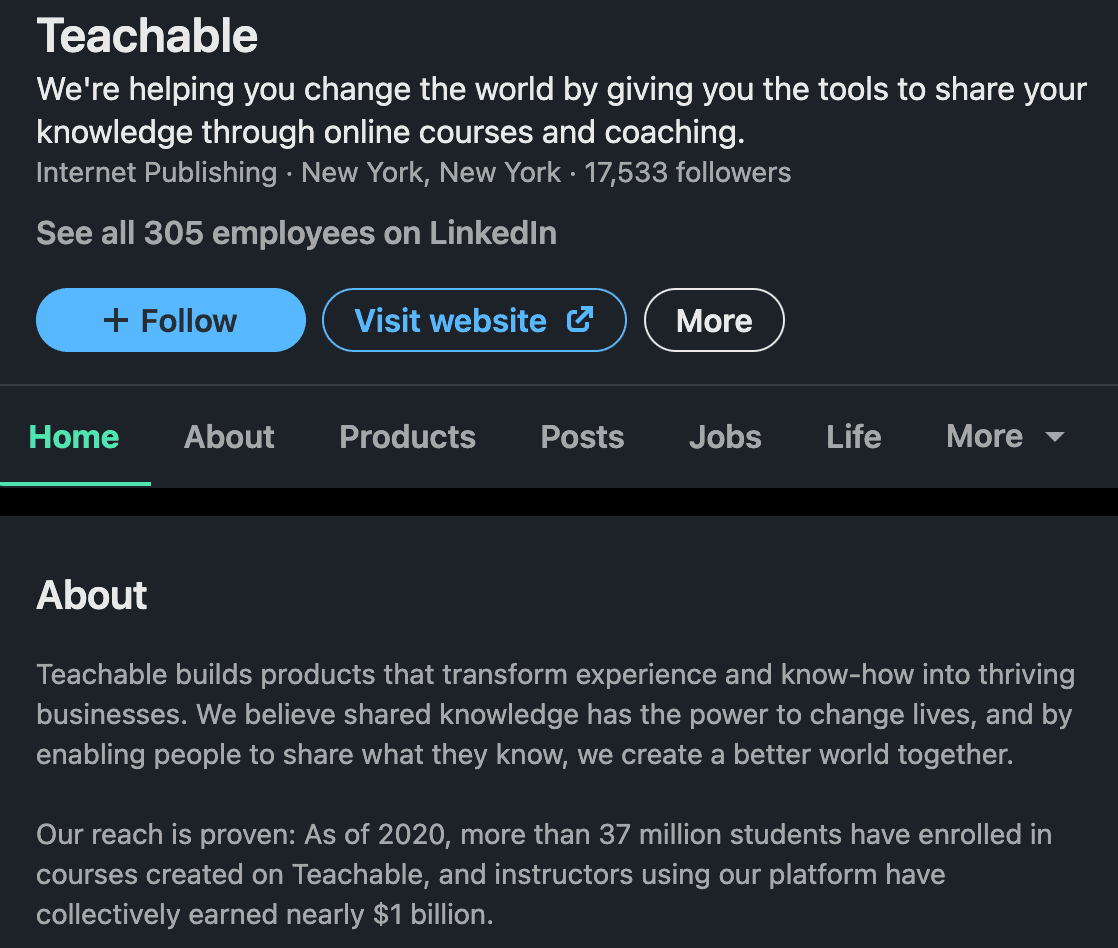The caption should read:

"An image displaying white text on a black background, featuring the title 'Teachable' at the top. Below the title, a descriptive sentence explains, 'We're helping you change the world by giving you the tools to share your knowledge through online courses and coaching.' This is followed by a descriptor stating, 'Internet Publishing, New York, New Yorker, 17,533 followers,' with an option to 'See all 305 employees on LinkedIn.' Beneath this, there are three buttons: a blue 'Follow' button, a black 'Visit Website' button with blue text, and a 'More' button. Additionally, seven tabs are visible: Home, About, Products, Posts, Jobs, Life, and More. The 'More' tab can be expanded by clicking a downward-pointing triangle. Currently, the 'About' section is selected, displaying two paragraphs of text below."